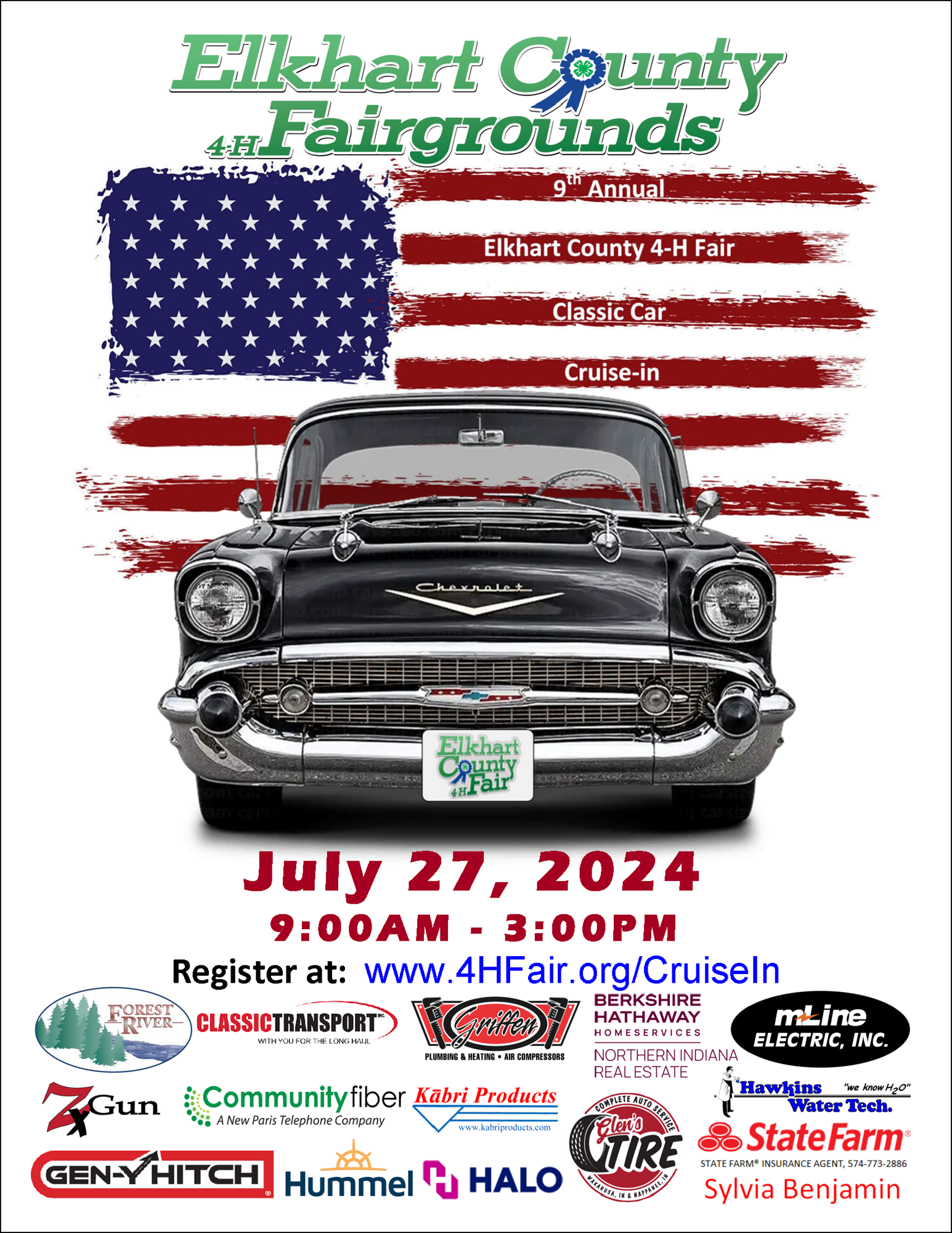The poster for the 9th Annual Eckhart County 4-H Fair Classic Car Cruise-In is set against a white background. At the top, "Eckhart County Fairgrounds" is prominently displayed in green letters. Below, a painted image of the American flag features artistic brushstroke edges, detailing the red stripes and the blue square with white stars. Within the red stripes of the flag, white letters announce the event details: "9th Annual Eckhart County 4-H Fair Classic Car Cruise-In." A vintage black Chevrolet car from the 1950s, showcasing round headlights, a silver grille, and a bumper, is prominently featured below the text. The event is scheduled for July 27, 2024, from 9 AM to 3 PM. Registration details are provided as "register at www.4hfair.org/cruise-in." At the bottom of the poster, various sponsor logos are displayed, including Glen's Tire, State Farm, M Line Electric Inc., Berkshire Hathaway, Hummel, Sylvia Benjamin, and Northern Indiana Real Estate.